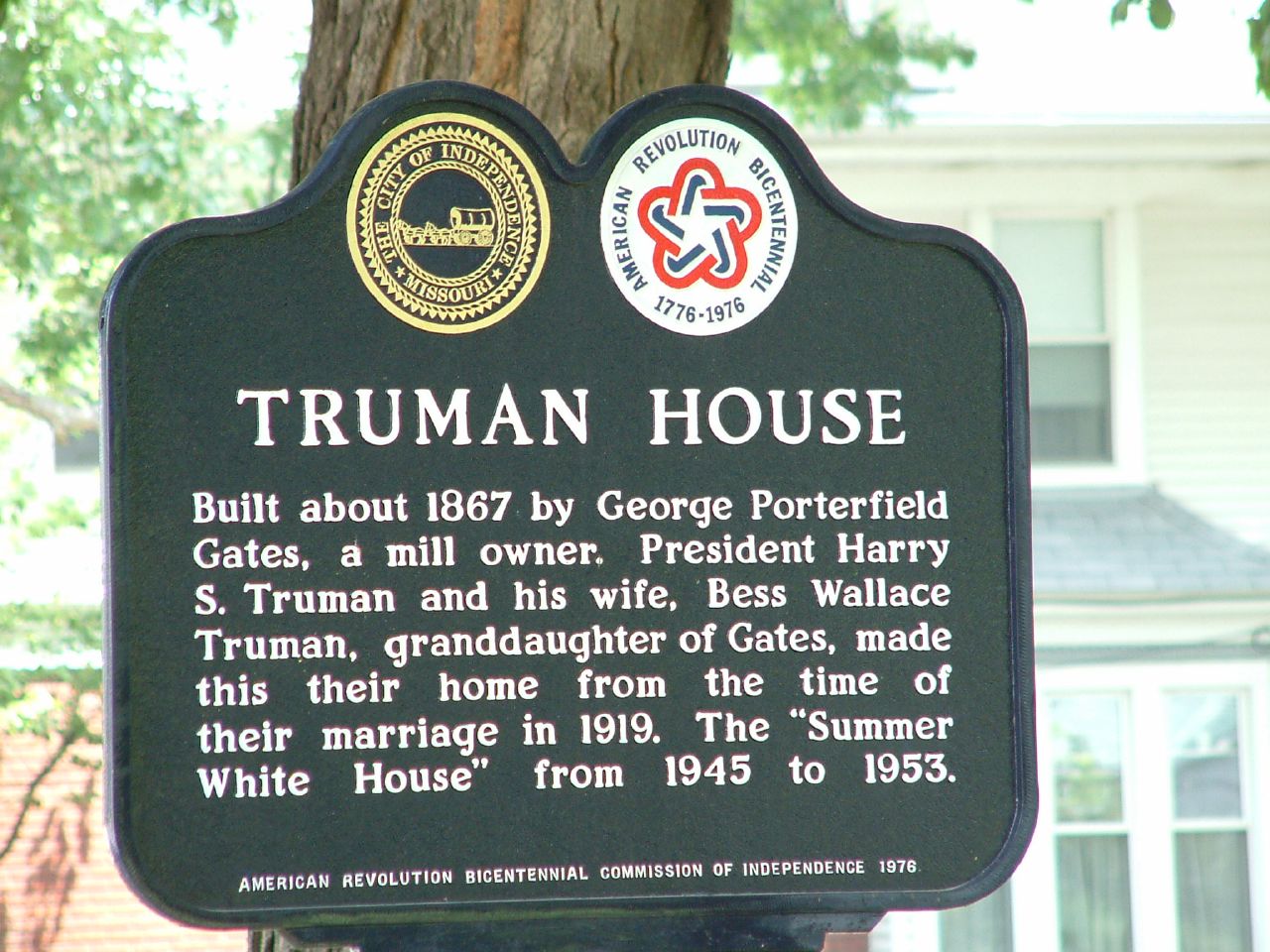The image captures a distinctive landmark sign in front of a tree, with a house faintly visible in the background during daylight. The black sign has a unique, rounded rectangle shape with two half circles at the top, featuring logos. On the left, the golden logo reads "City of Independence, Missouri," possibly showcasing a horse cart. On the right, a white logo with a red and blue five-sided star reads "American Revolution Bicentennial, 1776-1976." The main text on the sign, written in bold white lettering, declares "Truman House." Beneath it, in smaller white text, it states, "Built about 1867 by George Porterfield Gates, a mill owner. President Harry S. Truman and his wife, Bess Wallace Truman, granddaughter of Gates, made this their home from the time of their marriage in 1919, the Summer White House, from 1945 to 1953." At the bottom, in very small text, it notes, "American Revolution Bicentennial Commission of Independence, 1976." The overall setting showcases a historical marker amidst a serene, leafy environment with glimpses of the historic Truman House in the background.